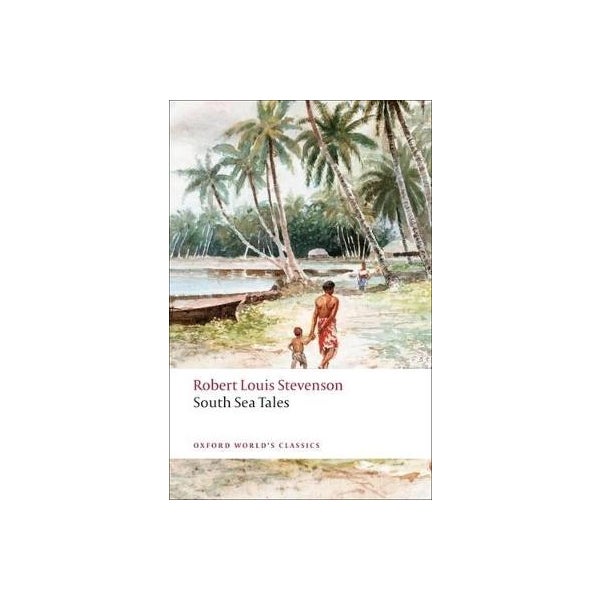The image depicts a book cover for "South Sea Tales" by Robert Louis Stevenson, part of the Oxford World's Classics series. The scene is a detailed illustration featuring a woman and a toddler, both seen from the back, holding hands as they walk along a brown dirt pathway. The path is set in a picturesque, tropical setting with lush green and brown hues, tall palm trees some of which are leaning over a small, green-tinged body of water on the left-hand side. There are also boats seen towards the side of the water, and a brown hut is faintly visible in the background among the trees. The sky is partly cloudy, adding to the serene yet slightly whimsical atmosphere. The title "Robert Louis Stevenson, South Sea Tales, Oxford World's Classics" is prominently displayed in a white horizontal banner at the bottom of the cover, with the main title in black and the series name in red. The overall composition and choice of colors give the image a painterly quality, integrating textual and visual elements seamlessly.